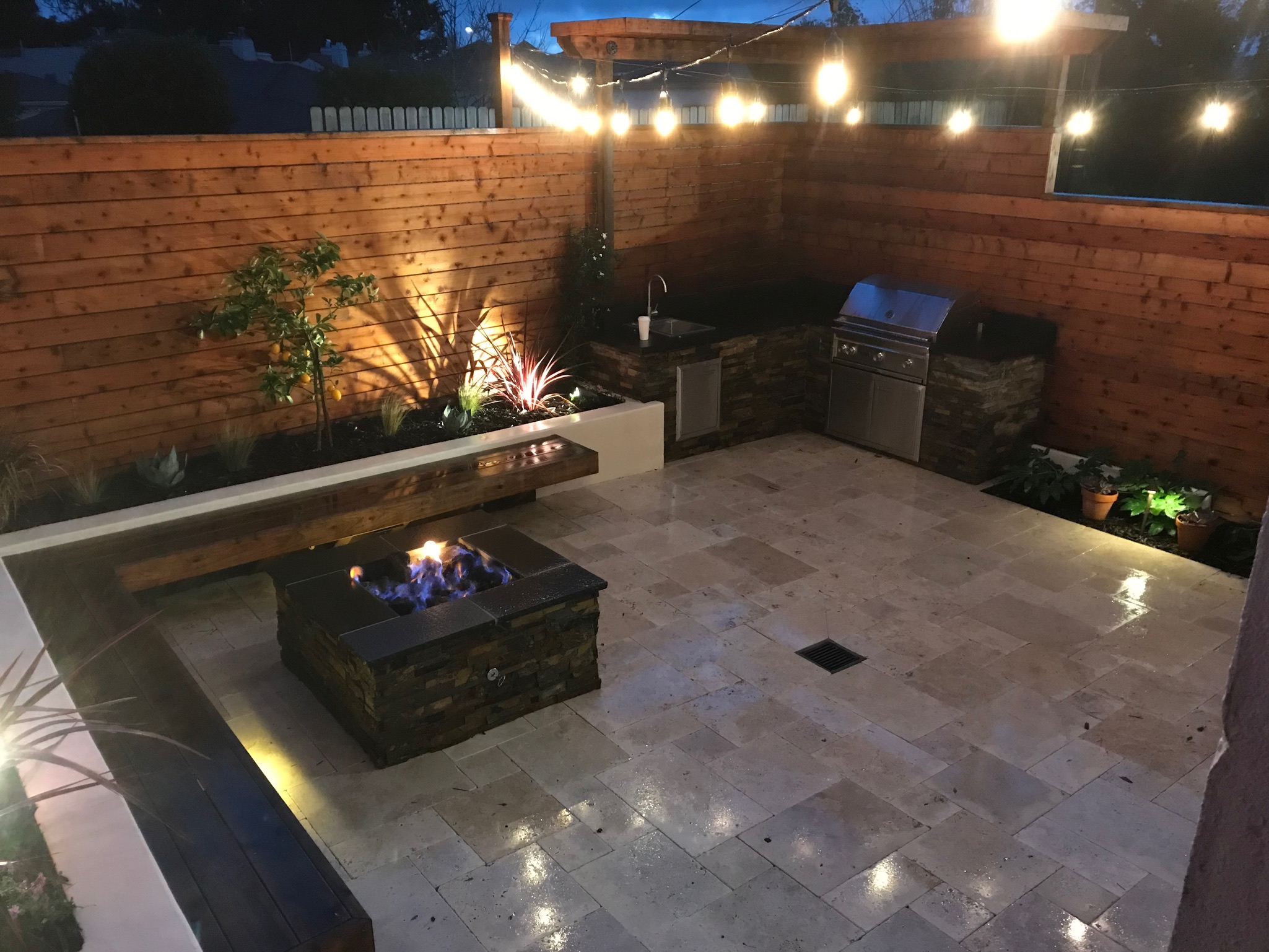The image depicts a beautifully arranged patio with an intricate floor composed of tightly-fitted square tiles, creating a seamless, light-colored surface. The patio is framed by wooden walls featuring light brown wood adorned with distinct knots. Hanging across the top of the patio is a string of yellow-colored light bulbs, casting a warm glow.

In the bottom left corner of the scene is a fire pit with a black stone surround. The fire pit features blue light within it and orange flames flickering above. Just to the left of the fire pit, there's a wooden bench backed by a white barrier, contributing to a comfortable seating arrangement. Surrounding the patio, various plants are visible; some grow behind the bench, and a small garden with potted plants is situated on the right side. Additionally, the right side hosts an outdoor cooking area, complete with a black outdoor grill, a sink, and counter space for food preparation. Adjacent to this setup is a water outlet with a fountain that arcs gracefully before descending back down.